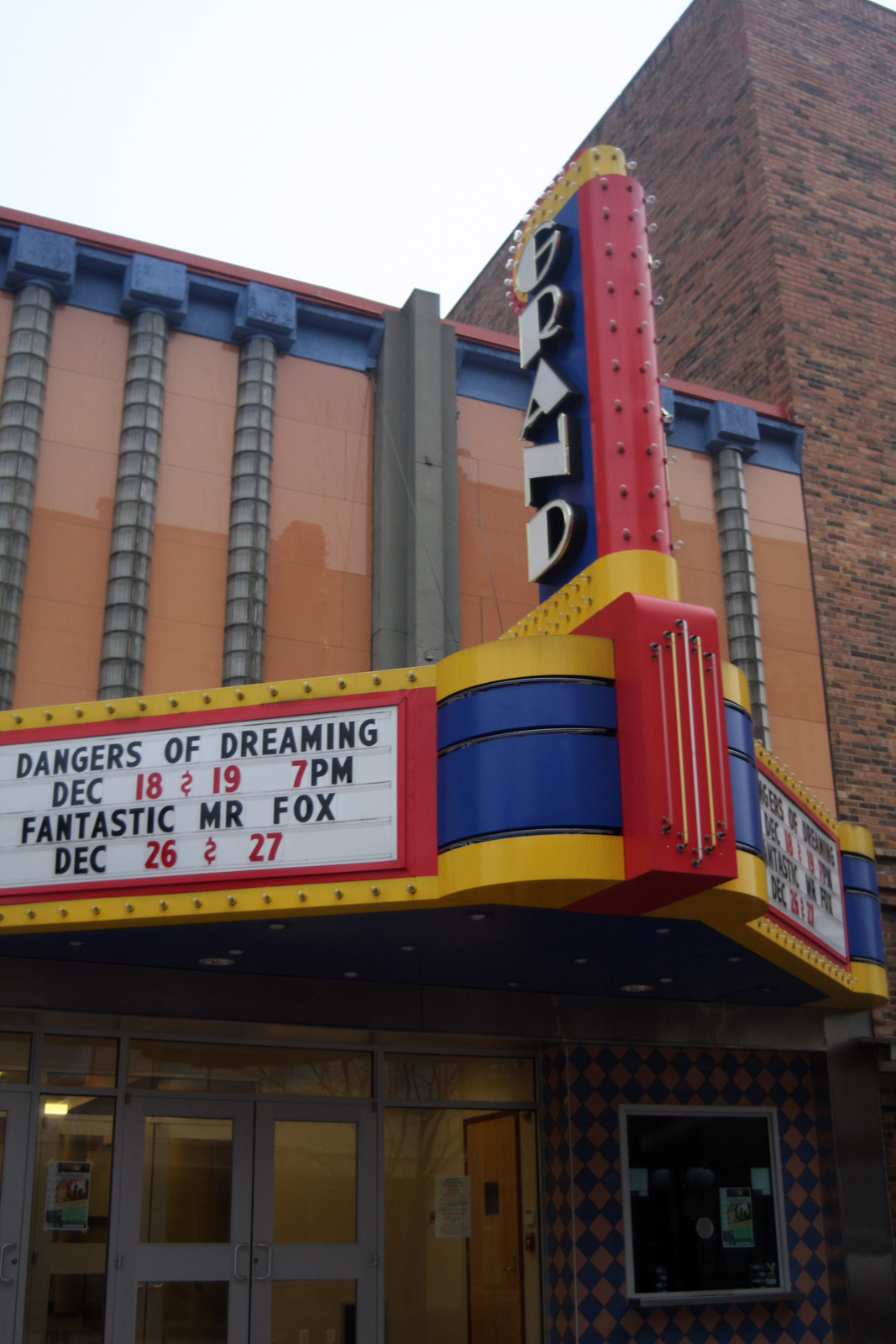The image showcases the front facade of The Grand Theater, a tall brick building partially attached to another structure on its right. Dominating the view, a vibrant marquee features "GRAND" in large, bold white letters oriented vertically. Below this marquee, details of upcoming shows are visible in colorful sections adorned with light bulbs, primarily in hues of red, yellow, and blue. The left marquee announces "The Dangers of Dreaming" on December 18th and 19th at 7 p.m., followed by "Fantastic Mr. Fox" on December 26th and 27th. It's likely that the right marquee mirrors these show details. The entrance area beneath the marquee includes darkly shaded double doors, which suggest evening lighting, though the scene occurs during the day, possibly under a cloudy sky. Adjacent to the entrance, on the right side, is a ticket kiosk window, seemingly closed, adding to the quiet, almost dormant atmosphere of the building. The overall aesthetic, with its ornate details and bright facade, offers an authentic and inviting feel for theatergoers.